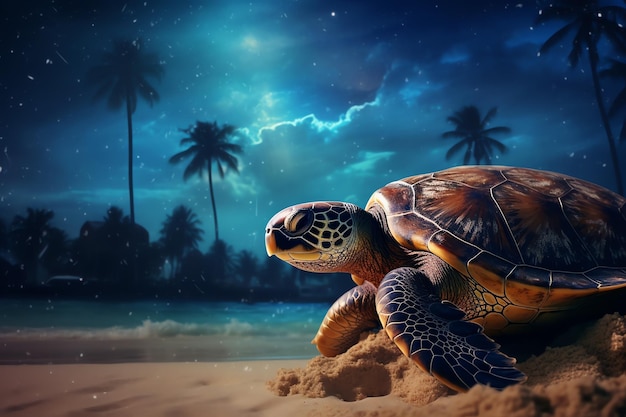This image is a highly detailed, illuminated nighttime painting capturing an artist's interpretation of a sea turtle on a beach under the moonlight. Dominating the foreground, the turtle, with its head facing left, showcases meticulously rendered dark brown flippers striped with white lines, a similarly colored shell with brown and white streaks, and an orange underside. Its face mirrors the pattern of the flippers, contributing to its vibrant presence. The turtle is depicted pushing through a brownish-beige mound of sand.

Stretching beyond the turtle, the scene transitions into a green, wave-flecked body of water, leading the eye to a silhouetted coastline adorned with palm trees and lower foliage. The sky above is a beautiful blend of green and aqua blue hues, interspersed with white clouds through which either the moon or the sun shines softly, casting a gentle, ethereal glow over the water and landscape. The overall ambiance evokes the serene beauty of a narrow waterway in Florida or the Caribbean, combining photorealistic detail with an air of digital artistry.